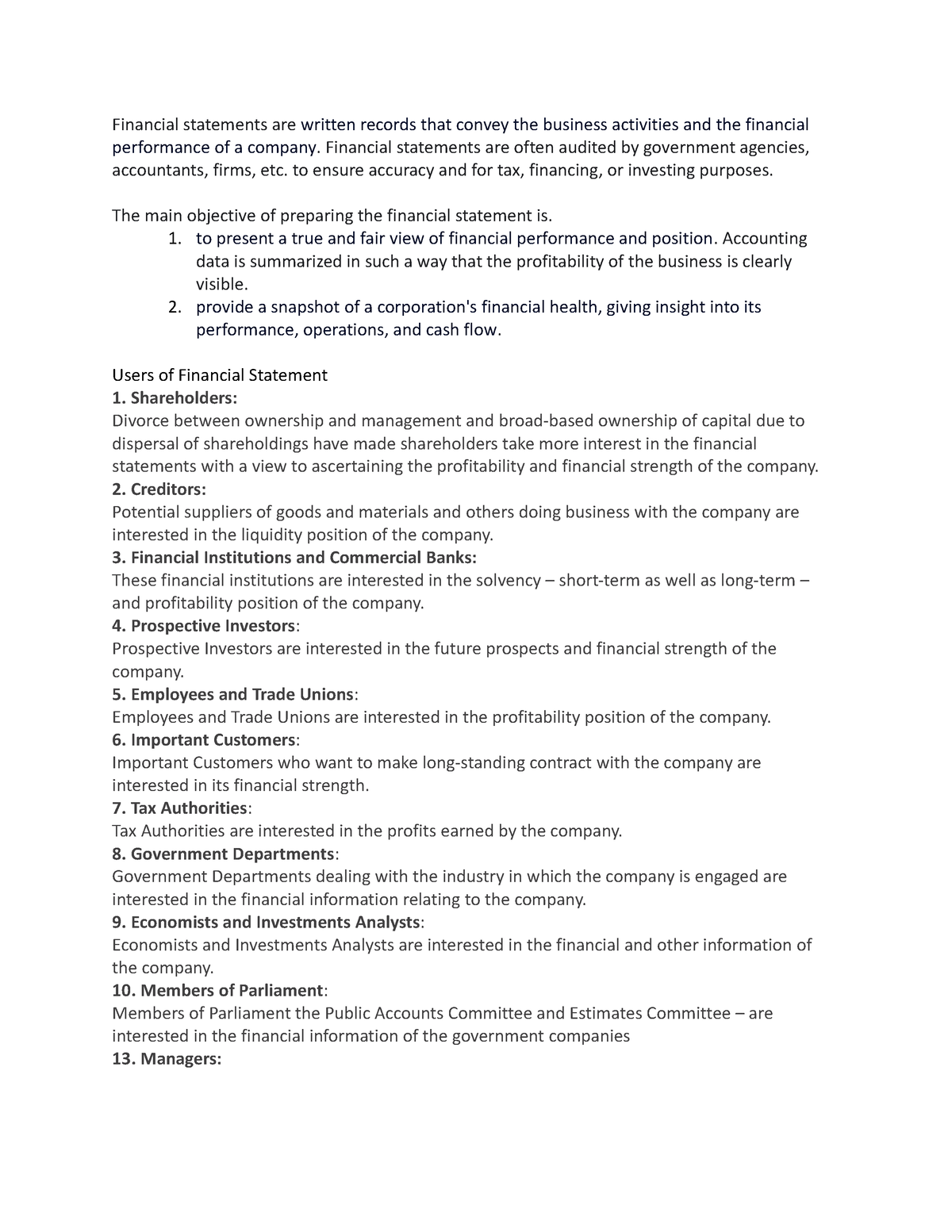The image displays a white page with meticulously organized black text detailing the concept and objectives of financial statements. The text explains that financial statements are written records that reflect the business activities and financial performance of a company. These documents are often audited by government agencies, accountants, and firms to ensure their accuracy for purposes related to taxation, financing, and investing.

The main objective of preparing a financial statement is highlighted, emphasizing its role in presenting a true and fair view of the company's financial performance and position. The accounting data is summarized to clearly display the company's profitability.

Additionally, the text outlines another key objective: to provide a snapshot of a corporation's financial health, offering valuable insights into its performance, operations, and cash flow.

A separate section is dedicated to the users of financial statements, listing 13 different users along with explanations for each. However, it's noted that the portion labeled "Managers" at number 13 lacks further details or explanations.